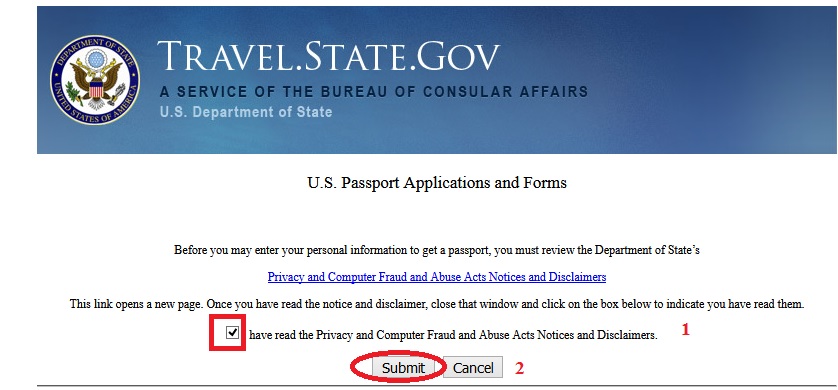The banner features a prominent blue rectangle at the top with bold white text that reads "travel.state.gov". Below this, there is additional text stating "A service of the Bureau of Consular Affairs U.S. Department of State". On the left side of the text, there is a circular emblem outlined in blue, with the words "Department of State United States of America" encircling the U.S. State Department seal. The seal showcases an eagle with outstretched wings, clutching various objects in its talons, and a flag at its center.

Beneath this segment, a header in black text on a white background announces "U.S. Passport Applications and Forms". Additional text follows below, some portions of which are blue and underlined, suggestive of hyperlinks. Additionally, there is a marked checkbox enclosed in a red rectangular or square border.

At the bottom of the banner, there are two buttons labeled "Submit" and "Cancel". The "Submit" button is circled in red, with the number "2" positioned nearby. Similarly, the checkbox is accompanied by the number "1".